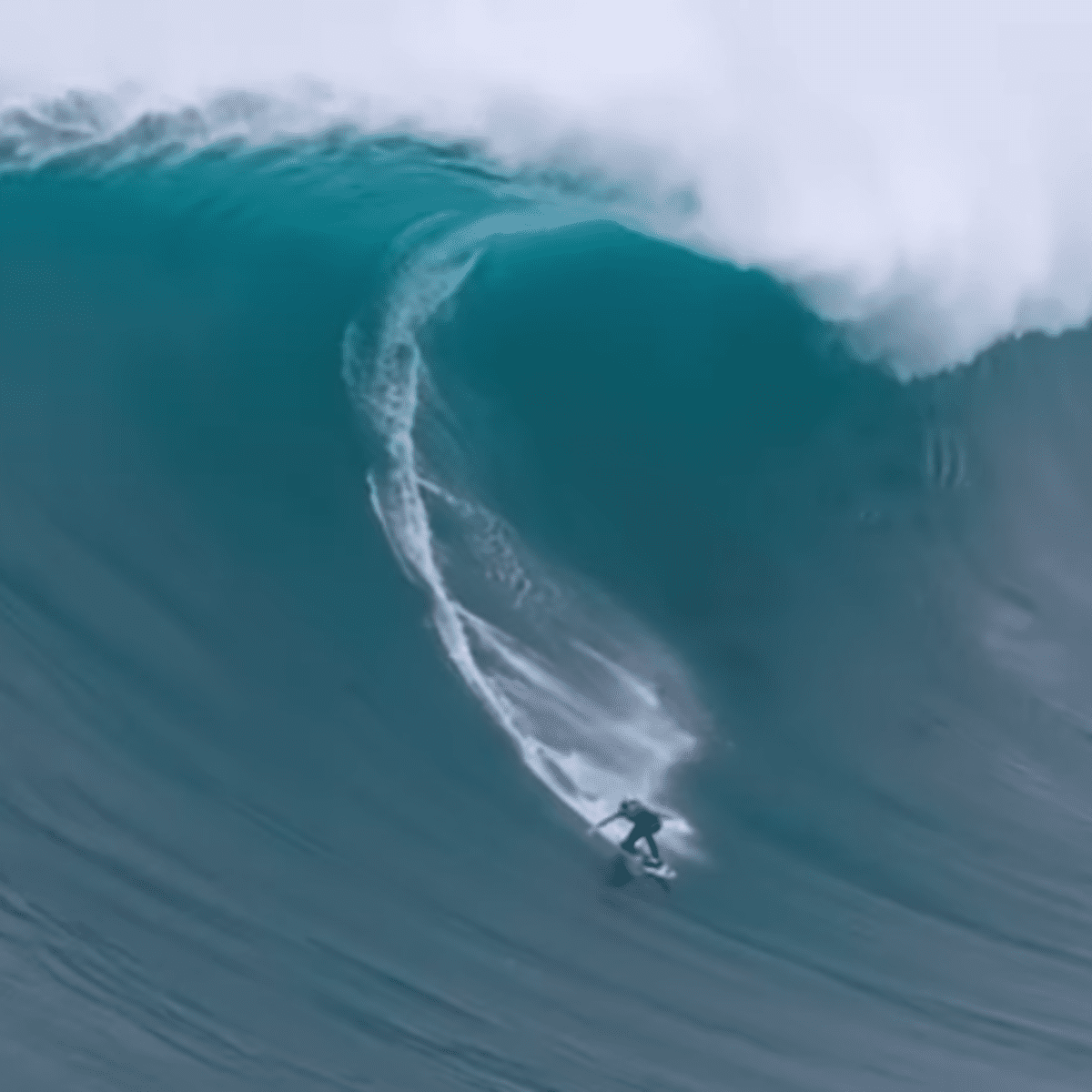This photograph captures an awe-inspiring, enormous wave dominating the entire frame with its dark bluish-green hues. The wave's towering presence is accentuated by its sharp contrast against the relatively small surfer near the bottom center of the image. At the top, the wave arches over and begins to crash, displaying a foamy white crest. The surfer, wearing a black wetsuit, skillfully navigates this colossal wave with arms outstretched for balance, one arm slightly in front and one towards his back. His knees are slightly bent and his body leans forward, eyes focused downward and to the right. Behind him, a white streak of disturbed water marks his swift trail. The sheer scale of the wave compared to the surfer emphasizes the immense challenge he's undertaking, and the out-of-focus effect on the wave further enhances the dramatic and somewhat surreal quality of this breathtaking scene.